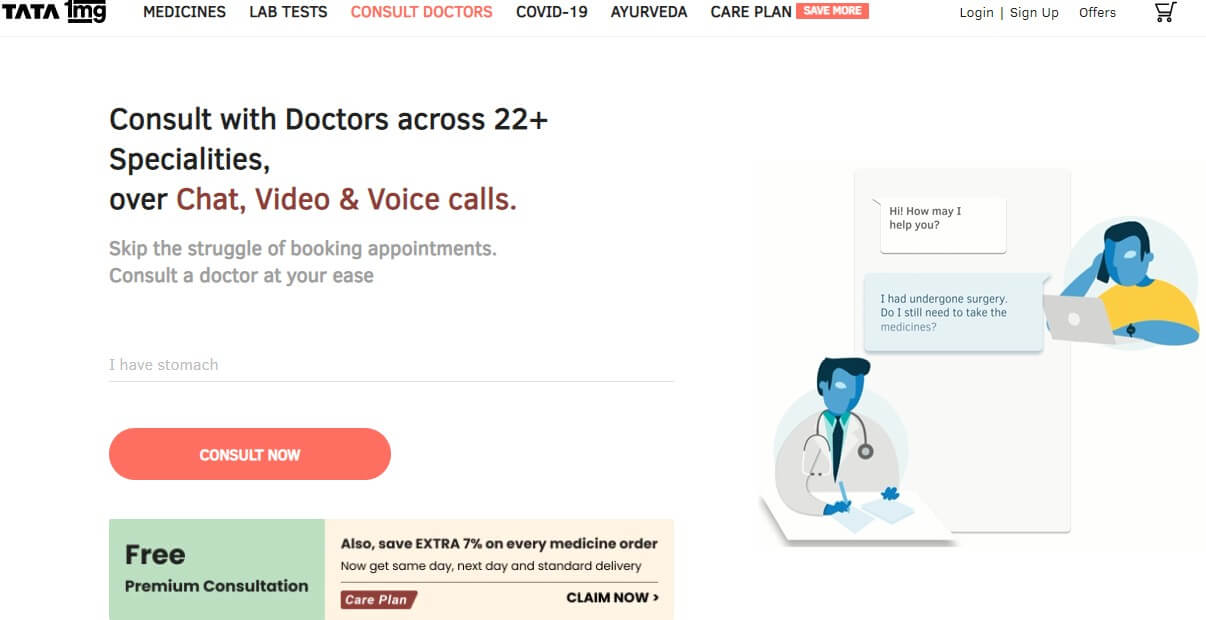The image appears to be an advertisement or a promotional section of a medical assistance website named "TATA." At the top of the page, there is a navigation menu with several tab options: "Medicines," "Lab Tests," "Consult Doctors" (which is highlighted in red), "COVID-19," another unspecified option, and "Care Plan." Additional options for "Log In," "Sign Up," and "Offers" are also available.

Below the menu, there is a prominent message in large bold black lettering that reads, "Consult with doctors across 22+ specialties." This is followed by text in red, stating "Chat, video, and voice calls." Further down, the message continues, "Skip the struggle of booking appointments, consult a doctor at your ease." 

A red clickable button with white lettering that says, "Consult Now," is prominently displayed beneath this message. To the right of this button, there are vector illustrations: one depicts a patient on the phone looking at a laptop, and another shows a doctor writing a prescription at a desk, adding a visual context to the services offered.